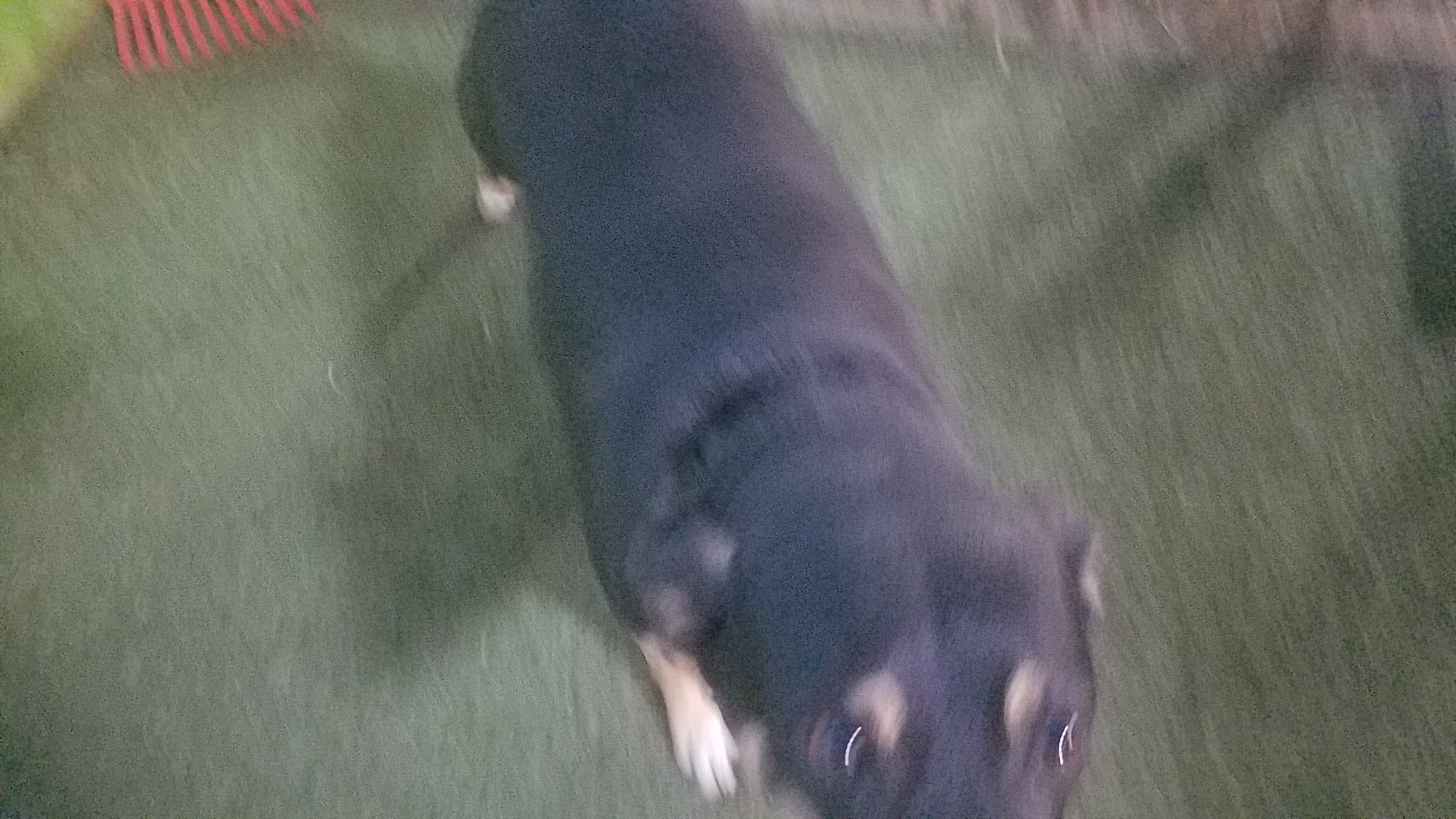The photograph features a predominantly black dog with tan and beige markings, specifically on its feet and spots above its eyes, standing on what appears to be grass or astroturf. The image is quite blurry, suggesting that either the dog or the photographer was in motion when it was taken. The dog’s snout is cut off, but its eyes, adorned with light brown eyebrows, are visible. While the exact breed is unclear due to the blurriness, it resembles a mix and has been described as potentially being a Pitbull, Rottweiler, Doberman Pinscher, or dachshund. A red rake's bristles are visible in the background. The photograph is shot from above in a wider-than-tall format, emphasizing the dog's long body, which adds to the blurry dynamic composition.